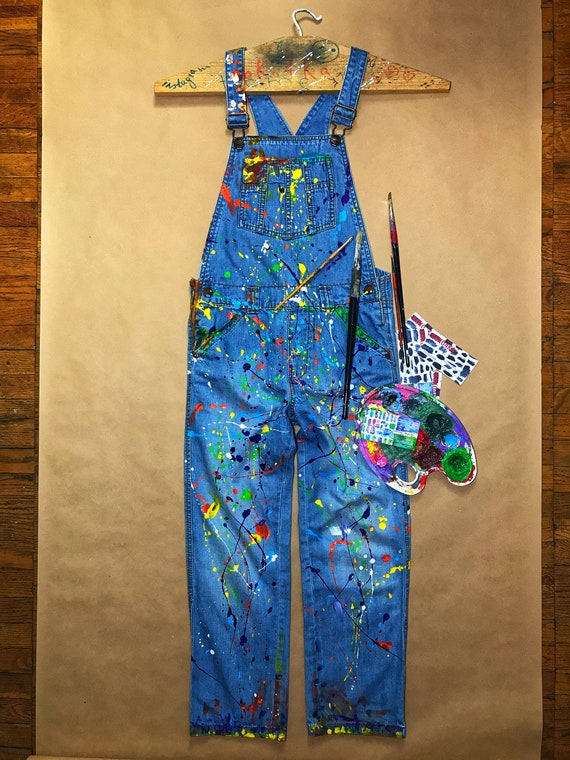This image presents a meticulously arranged bird's eye view of a painter's workspace against a rich brown-orange hardwood floor. Centrally displayed on a large sheet of brown butcher paper is a pair of well-worn denim overalls, suspended from a solid wooden hanger that features an assortment of hand-drawn faces, shapes, and paint splatters. The overalls, intact and richly speckled with an array of paint colors—including vibrant hues of red, blue, green, yellow, orange, black, and white—suggest significant use by a dedicated artist. 

To the left of the overalls lies a well-used artist's palette, brimming with a kaleidoscope of mingling colors, a testament to the creative process. Scattered around and atop the overalls are several paintbrushes of varying sizes and colors, some with paint still visible on their bristles, and a few small pieces of paper bearing signs of color testing. Together, these elements evoke a vivid scene of artistic endeavor, poised in anticipation of the next splash of creativity.